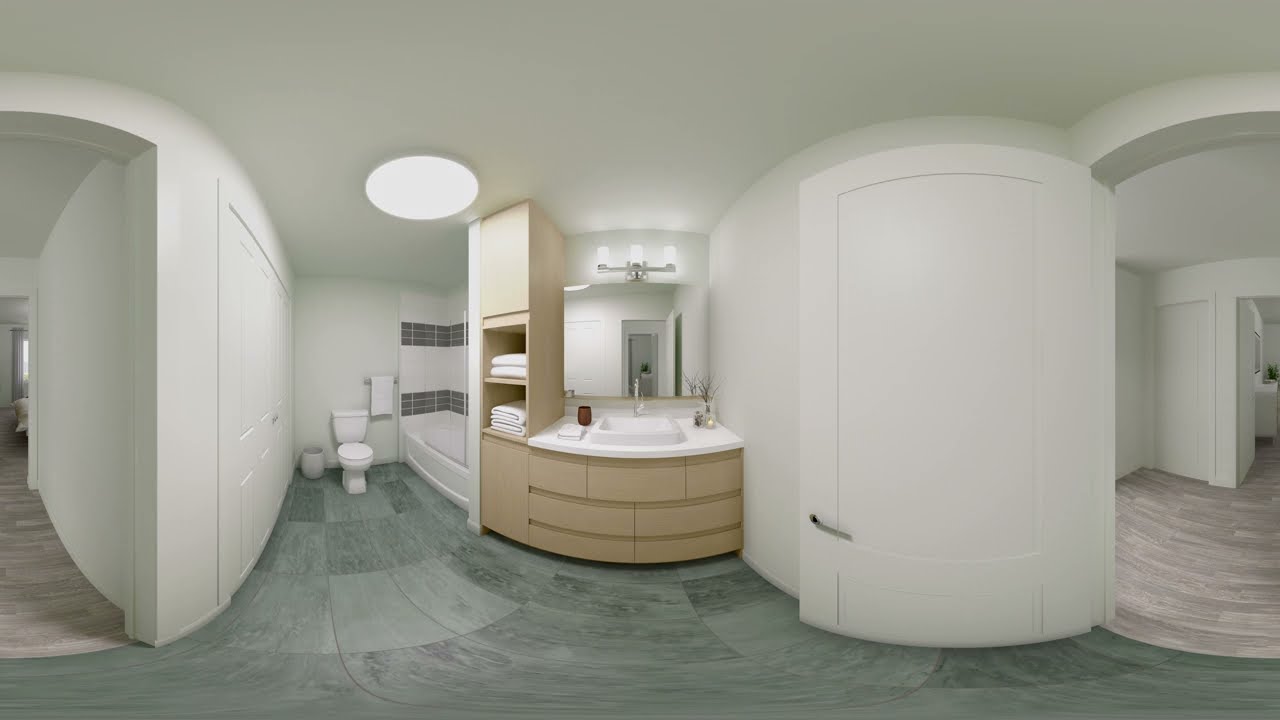This detailed image captures an immaculate, indoor bathroom with a pristine, white ceiling and walls. The floor boasts a marble-effect tile in a sophisticated mix of blue and gray tones. At the room's center lies a white countertop with an integrated sink, flanked by light brown cabinets that contain neatly arranged white towels. Adjacent to the vanity is a streamlined white bathtub adorned with dual rows of either gray or blue horizontal tiles. A single white towel hangs on a rack next to the tub. Positioned to the left, near the bathtub, is a standard white toilet accompanied by a small trash can. Notably, the image also reveals two adjacent rooms, visible through open doorways that lack doors and feature lighter wood flooring and white walls. Above the vanity, a light fixture illuminates the space, and a glass mirror complements the clean aesthetic. Additionally, a distorted bubble effect in the photo warps the edges, making elements like a closed door appear curved, even though they are straight in reality.